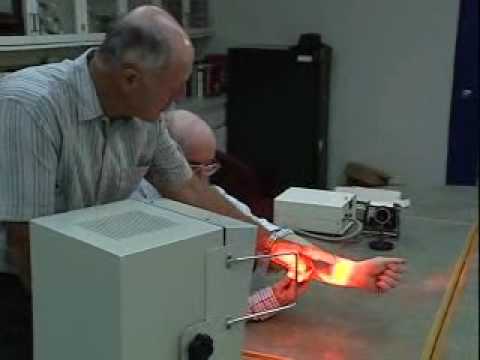In this photograph, two middle-aged men, resembling professors, engineers, or scientists, are immersed in a laboratory experiment. The man seated on the left is wearing glasses and is faced by another man standing in the foreground, who is bald on top and dressed in a pinstripe shirt with a white collar. They are both positioned around a large table cluttered with various instruments. Central to their focus is a contraption on the table emitting a very bright light, which is illuminating the inside of their forearms. The standing man's skin glows with bright shades of yellow and orange. Beside this light-emitting device, additional technology is present, including an old-fashioned computer, a camera with a prominent lens, and several grey boxes likely associated with the experiment. The backdrop reveals an office or lab setting with black filing cabinets, a door, and windows along the wall to the left. They both gaze intently at the light and their arms, deeply engrossed in their scientific endeavor.